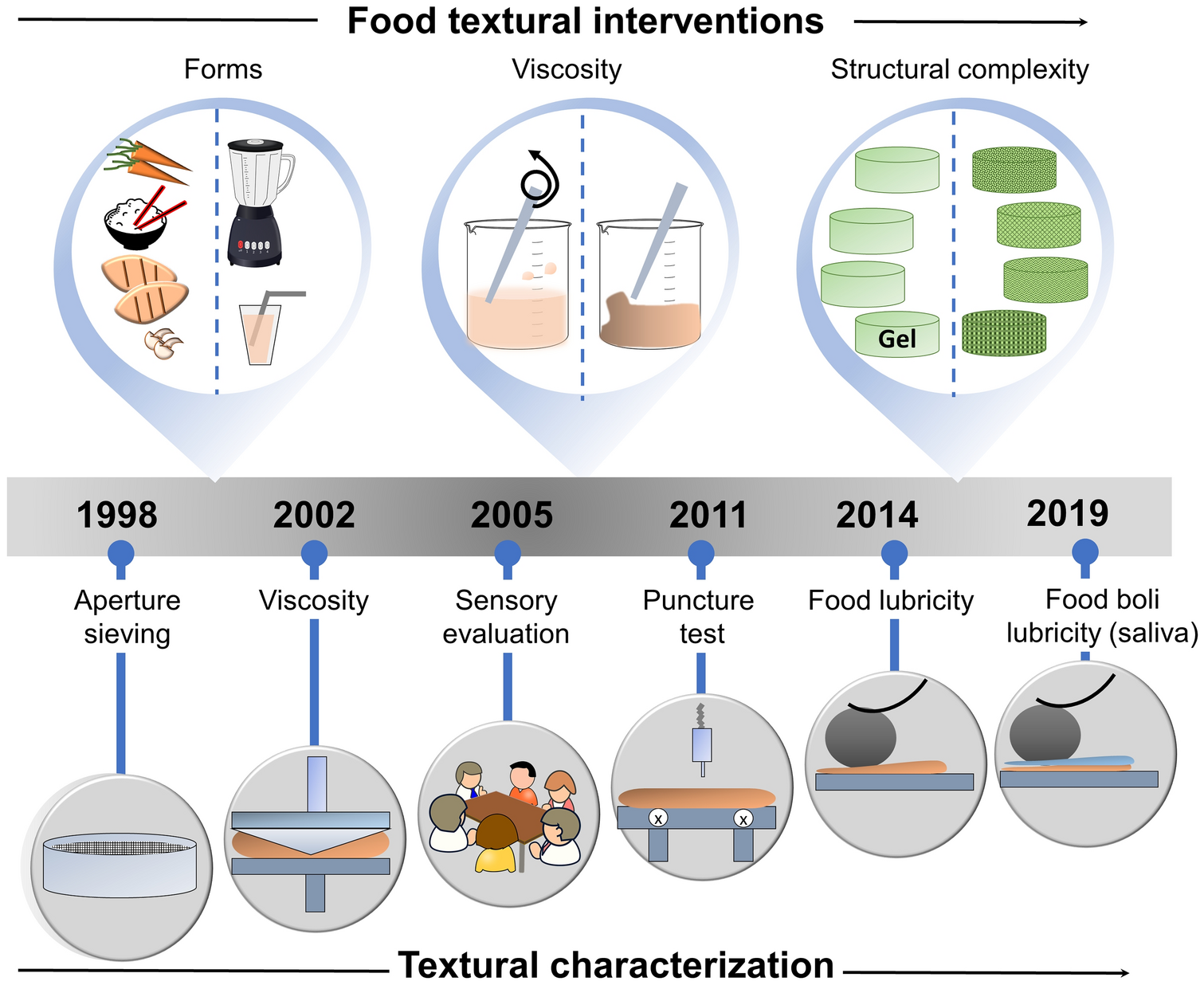The diagram, titled "Food Textural Interventions," presents a timeline from 1998 to 2019, highlighting key breakthroughs in food texture evaluation. Above the timeline, three interconnected sections detail different aspects of food texture. On the far left, labeled "Forms," the graphic showcases various kitchen items, including a blender, a glass with a straw, carrots, a bowl of rice with chopsticks, chicken breasts, and mushrooms. Adjacent to this, the "Viscosity" section displays two beakers with liquids and stir sticks. The final section, "Structural Complexity," features green disks labeled "gel."

Below the timeline, under the heading "Textural Characterization," the diagram lists six major milestones with corresponding diagrams: 
- 1998: Aperture sieving 
- 2002: Viscosity 
- 2005: Sensory evaluation (with a picture of a family)
- 2011: Puncture test 
- 2014: Food lubricity 
- 2019: Food boullion lubricity (saliva)

Each milestone is visually represented, underscoring the progression and refinement of techniques used in food texture assessment over the years.